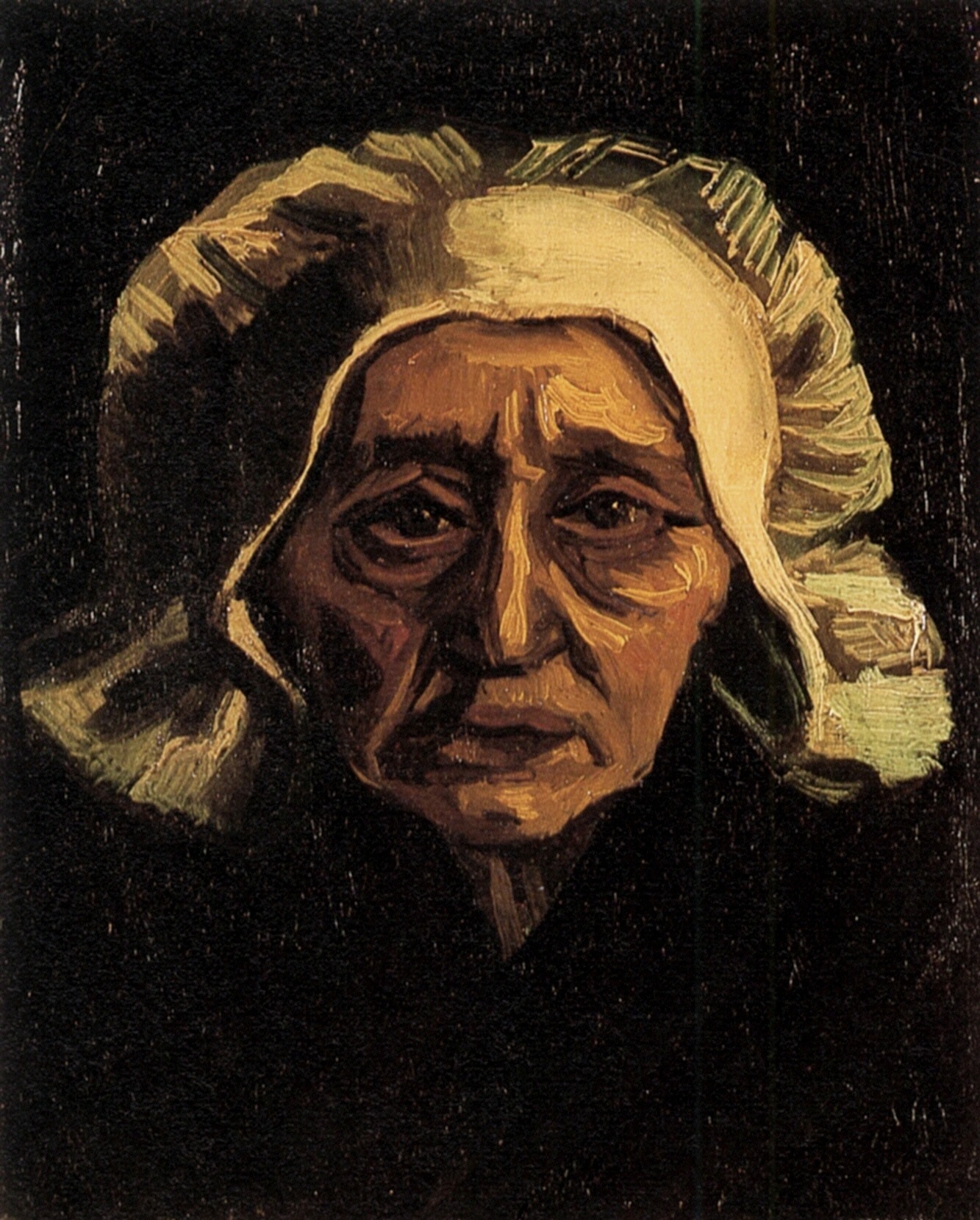This is an up-close oil painting of an elderly Native American woman, set against a predominantly black background with subtle white speckling. The focus is entirely on her worn and weary face, etched with deep wrinkles around her eyes, mouth, and forehead. Her large, dark brown eyes, filled with a troubled and pained expression, stare out from the canvas, conveying a profound sense of anguish. Her mouth is set into a sorrowful frown, further accentuating her distressed demeanor. She is depicted wearing a cream-colored bonnet that floats away from her ears and the top of her head, contributing to the image's striking visual impact. The light source in the painting highlights the textured brush marks on her dark skin, adding a palpable sense of depth and realism to her character. Only a small triangle of her neck is visible beneath her chin, with the rest of her figure dissolving into the black void that surrounds her.